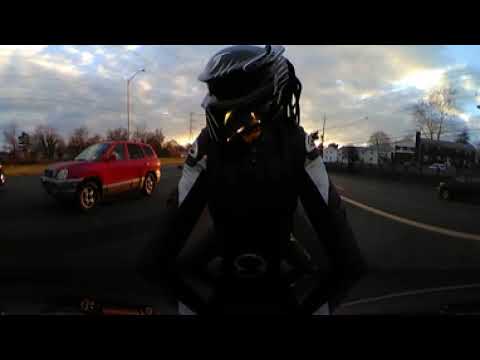This detailed image captures a close-up from the rear of one or possibly two motorcyclists adorned in black with distinctive white shoulder pads. The rider sports a striking black helmet, adorned with unique squiggles, perhaps resembling flames. The scene is likely viewed from a car's back window, where the motorcyclist is stationary, possibly waiting in line, suggested by the presence of a red car approaching from the left side and another vehicle either parked or merging from the right. The backdrop features a sparse arrangement of houses and leafless trees, signifying a less densely populated area. The cloudy, dusk sky dominates the upper third of the image, lending a somber, overcast atmosphere. Two black bands frame the image on the upper and lower horizontal edges, enhancing its cinematic feel.